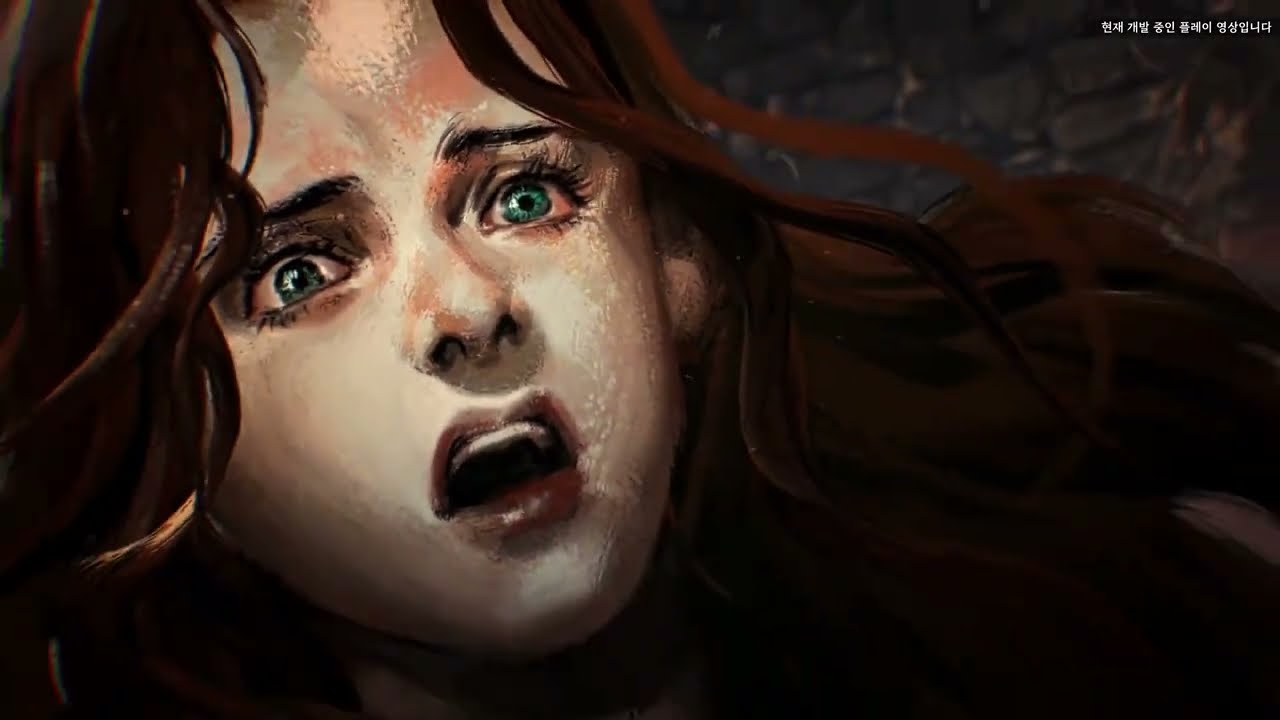The image resembles a highly detailed painting or illustration with a dark, eerie atmosphere. It prominently features a young woman with light, tan skin that's shinier around her nose and mouth. She has long, wavy auburn hair and striking green-blue eyes wide with terror, appearing to scream or in a state of shock. Her mouth is slightly open, showing red lips and white teeth against a dark backdrop inside her mouth. The woman occupies a significant portion of the left side of the image, which showcases her face and part of her neck, though the top of her head is cut off. She is looking upwards, seemingly reacting to something horrifying that is outside the frame.

The background includes dark gray bricks, suggesting a stone path or brick wall, and the setting appears to be dark or outdoors. The upper right corner contains some text in an East Asian script, possibly Korean or Japanese. The overall color palette includes shades of dark gray, black, white, brown, dark red, and various shades of green, enhancing the somber and frightening mood of the scene. The composition and details imply that something bad is about to happen to her, adding to the unsettling vibe of the image.